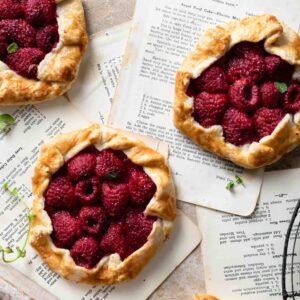In this beautifully arranged image, three circular raspberry pies are showcased, each boasting a golden-brown crust that frames a vibrant, red filling of fresh raspberries. The raspberries appear exceptionally fresh and juicy, enhancing the visual appeal of the pies. These delectable desserts are carefully placed on a table, atop scattered pages from a vintage black-and-white cookbook, creating a charming, rustic backdrop. The pies are thoughtfully positioned with one at the bottom center, one at the top right, and the last one at the top left, making a visually pleasing triangular formation. Each pie remains whole, uncut, and looks utterly delicious, with their perfectly baked crusts promising a delightful crunch.